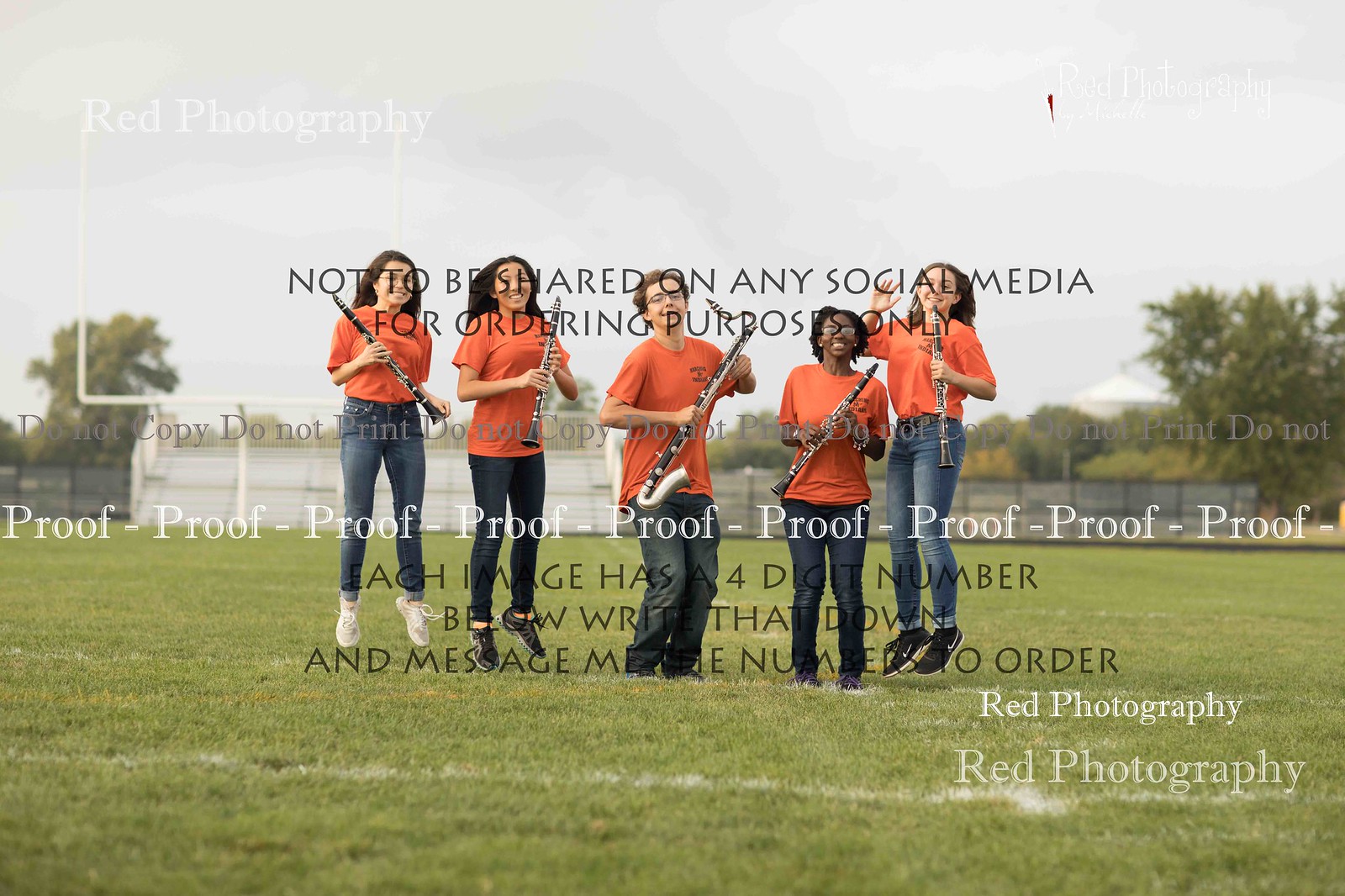This proof photograph from Red Photography, not to be shared on social media for ordering purposes only, features five young musicians leaping into the air on a cloudy day. They stand on what appears to be a football field, evidenced by the faint white stripes on the lawn and goalposts in the background. The backdrop includes lush green trees with hints of yellow and a set of bleachers. All five individuals are dressed in bright orange t-shirts and jeans, with some sporting black or white sneakers. Among them, a girl with darker denim jeans holds a clarinet and accessorizes with glasses, earrings, and bracelets on both wrists. Another notable musician in the center holds a saxophone. The photograph is clearly marked as a proof with watermarks from Red Photography and contains a four-digit identification number beneath each image.